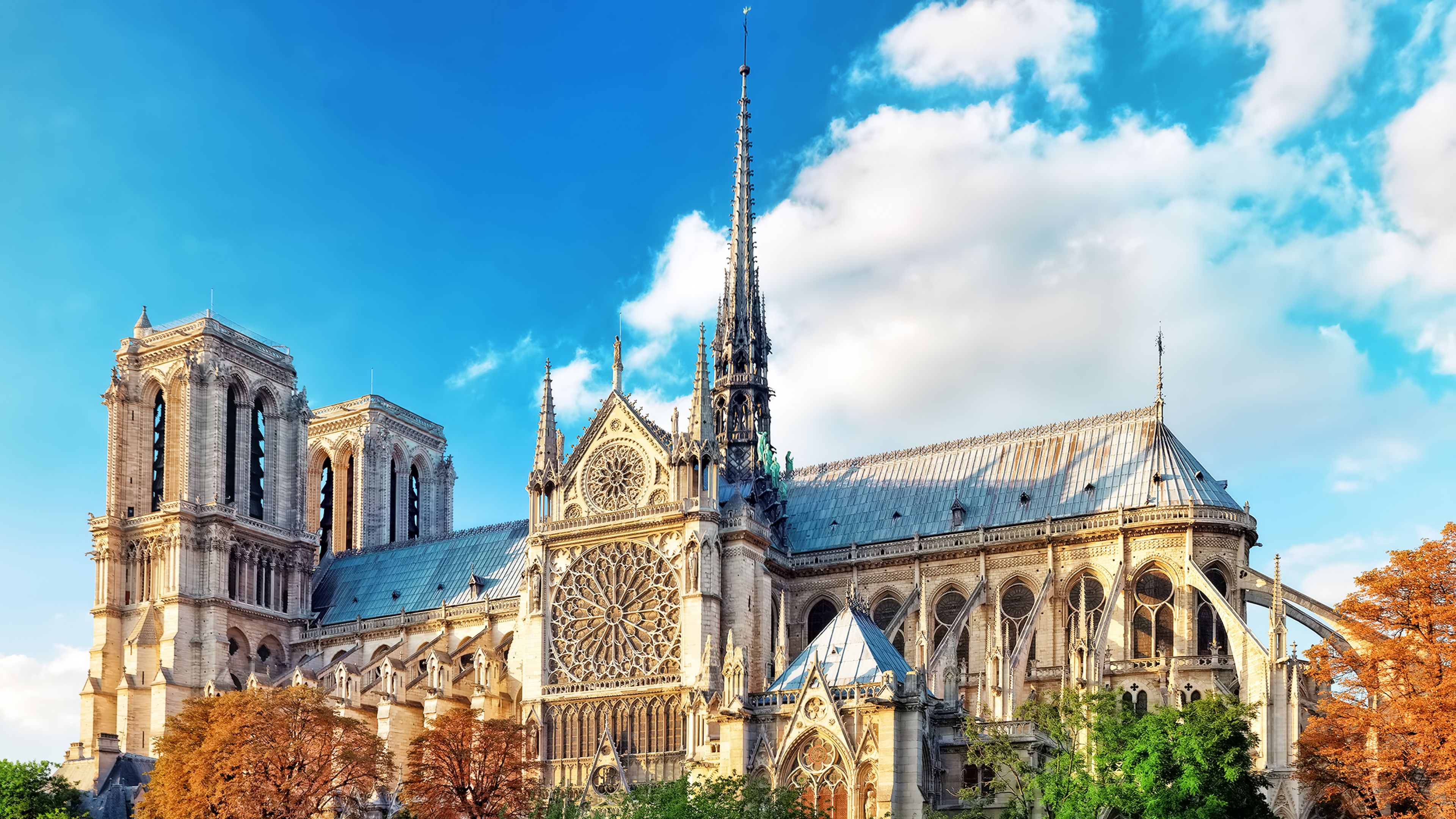The image depicts a colossal, ancient cathedral with distinctive old Italian architectural features, standing prominently in broad daylight under a bright blue sky. The cathedral's exterior is predominantly white, including its high, pointy steeples and large peaks. The central structure boasts a round geometrical shape that resembles a kind of clock, flanked by tall Roman-style columns, and the upper part of the building displays extensive window gaps that likely accommodate stained glass windows. The steeples house bells, and there are gargoyles adorning the structure.

Surrounding the grand cathedral are numerous tall trees, adding to the majestic sight. Of particular note, three of these trees exhibit a rich burnt orange color, suggesting it might be fall, while other trees, including one very green tree, add vibrant greenery to the scene. The sky above features a large cloud, contributing a dramatic backdrop to the splendid view of the cathedral.